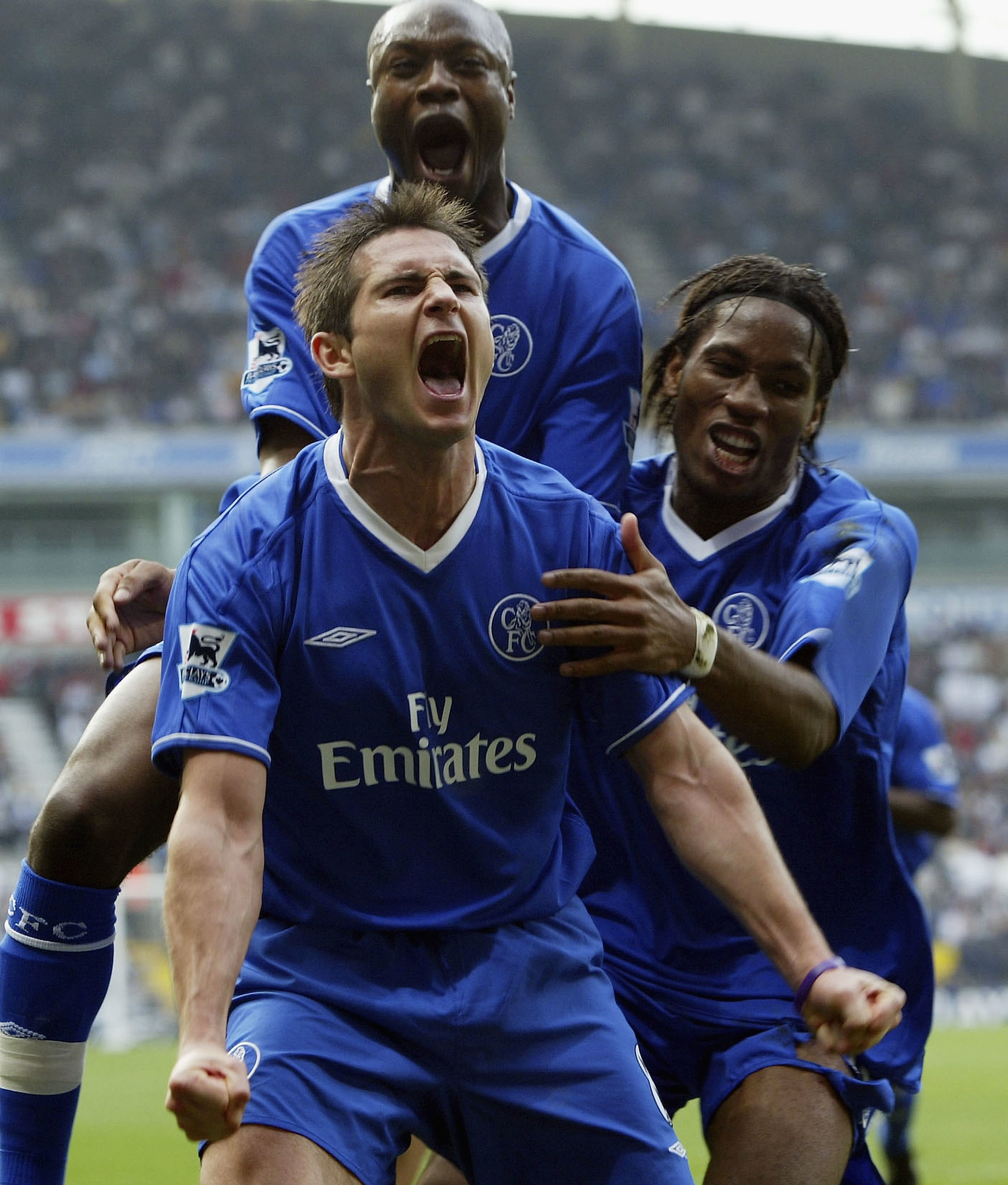In this vintage photograph, a youthful Frank Lampard, along with two jubilant African teammates, are seen celebrating a triumphant moment during a daytime soccer match. Lampard, who is the main focus, is elated, capturing the intense emotion of the scene. One of his teammates is caught mid-air in a joyous leap, while the other envelops him in a heartfelt embrace. All three players don the emblematic blue Chelsea jerseys, proudly displaying the Emirates sponsorship, the Barclays League logo, and the iconic Chelsea club crest. The background reveals a fully packed stadium, with the excited crowd slightly blurred, capturing the lively atmosphere. The edges of the grass pitch and part of the goalpost are also visible, grounding the image in a classic match setting.